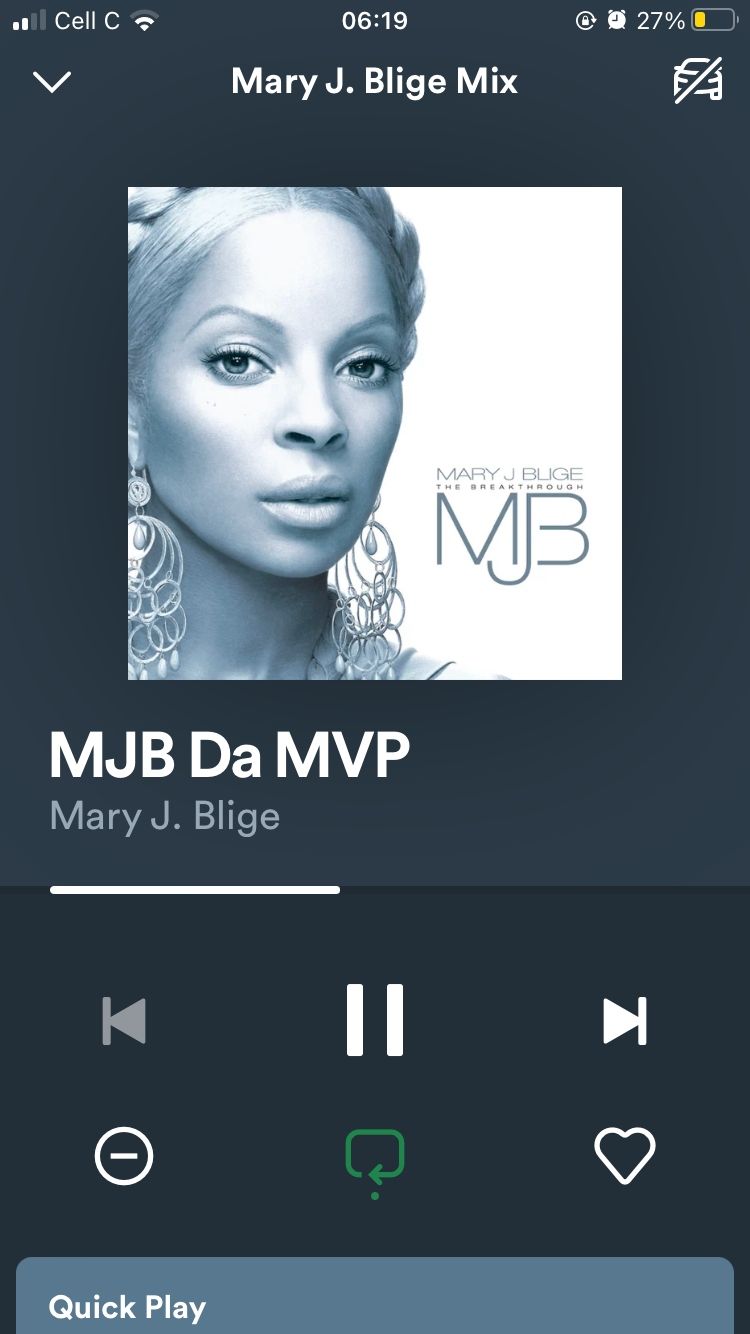Here is a highly detailed and cleaned-up caption for the described image:

---

This is a screenshot of a music application displayed on a cell phone. In the top left and right corners of the screen, typical cell phone icons are visible, indicating network status, battery life, and other notifications. The central focus of the screenshot is an album cover featuring a close-up image of Mary J. Blige. The album is titled "The Breakthrough," and this information is prominently displayed in bold white text within a white box. 

The photograph shows Mary J. Blige looking directly towards the camera, with her head slightly tilted to the right. Underneath the image, the initials "MJB" are shown in large white font, followed by "D-A M-V-B" – likely an artistic stylization. Directly underneath in smaller, gray font, the name "Mary J. Blige" is displayed. 

Towards the bottom of the screenshot, there's a white navigation bar providing controls for the music app. This bar includes a stop button in the center, flanked by a back button on the left and a forward button on the right, allowing users to navigate through tracks.

---

This caption encapsulates all elements of the screenshot with precise details, ensuring a clear understanding for any viewer.